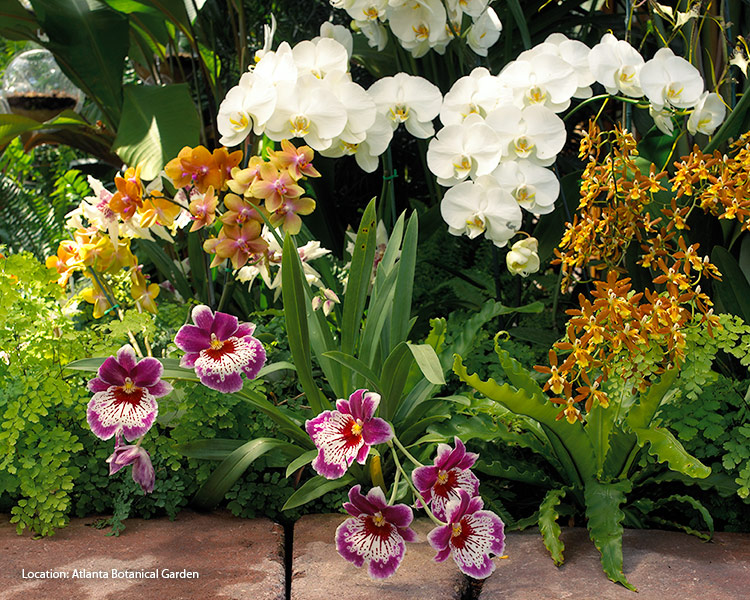This photograph captures a vibrant display at the Atlanta Botanical Garden. The array of flowers includes various types of orchids and other floral plants arranged in a visually striking manner. Dominating the top, center, and right are clusters of white orchids, some featuring delicate golden accents. The bottom, center, and left of the image showcase purple orchids with white centers, complemented by nearby darker golden orchids, which have subtle purple centers on the left and plain petals on the right. Interspersed among these colorful flowers, you can find smaller, clustered dark orange and light orange flowers toward the right, adding a dynamic mix. The scene is enriched with lush green foliage in the background and foreground, where stone or brickwork adds a structured feel to the natural beauty. The photograph is taken during the day, evident by the sunlight highlighting the detailed textures and colors of the plants. A text at the bottom left corner of the image identifies the location: Atlanta Botanical Garden.